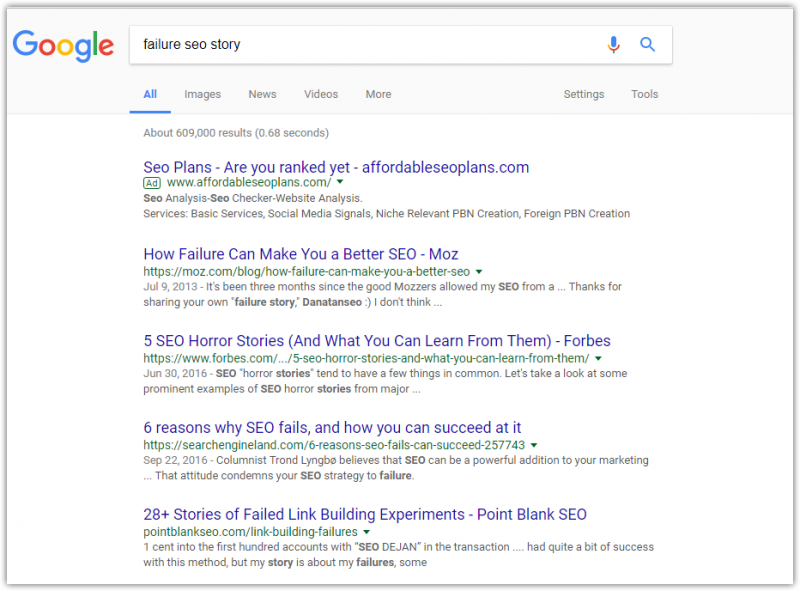The image depicts a Google search page. At the top left corner, the iconic Google logo is visible with its distinct colors: the "G" is blue, the first "O" is red, the second "O" is yellow, the second "G" is blue, the "L" is green, and the "E" is red. Centrally positioned at the top is the search bar. On the far left side of the search bar, the search query "Failure SEO Story" is typed in. Adjacent to this, on the right side of the search bar, are a microphone icon and a magnifying glass icon symbolizing voice search and search functionality respectively.

Just below the search bar, the navigation options "All," "Images," "News," "Videos," and "More" are listed horizontally. The word "All" is highlighted in blue, indicating it is the current selection, with a blue horizontal line beneath it. Farther right, "Settings" and "Tools" are displayed.

Further down, the search results are introduced with a note mentioning approximately 609,000 results. The first result is a link titled "SEO Plans, Are You Ranked Yet?" The second result is "Health Failure Can Make You A Better SEO." The third result reads "5 SEO Horror Stories." The fourth result is "6 Reasons Why SEO Fails." Lastly, the fifth result is "28 Plus Stories."